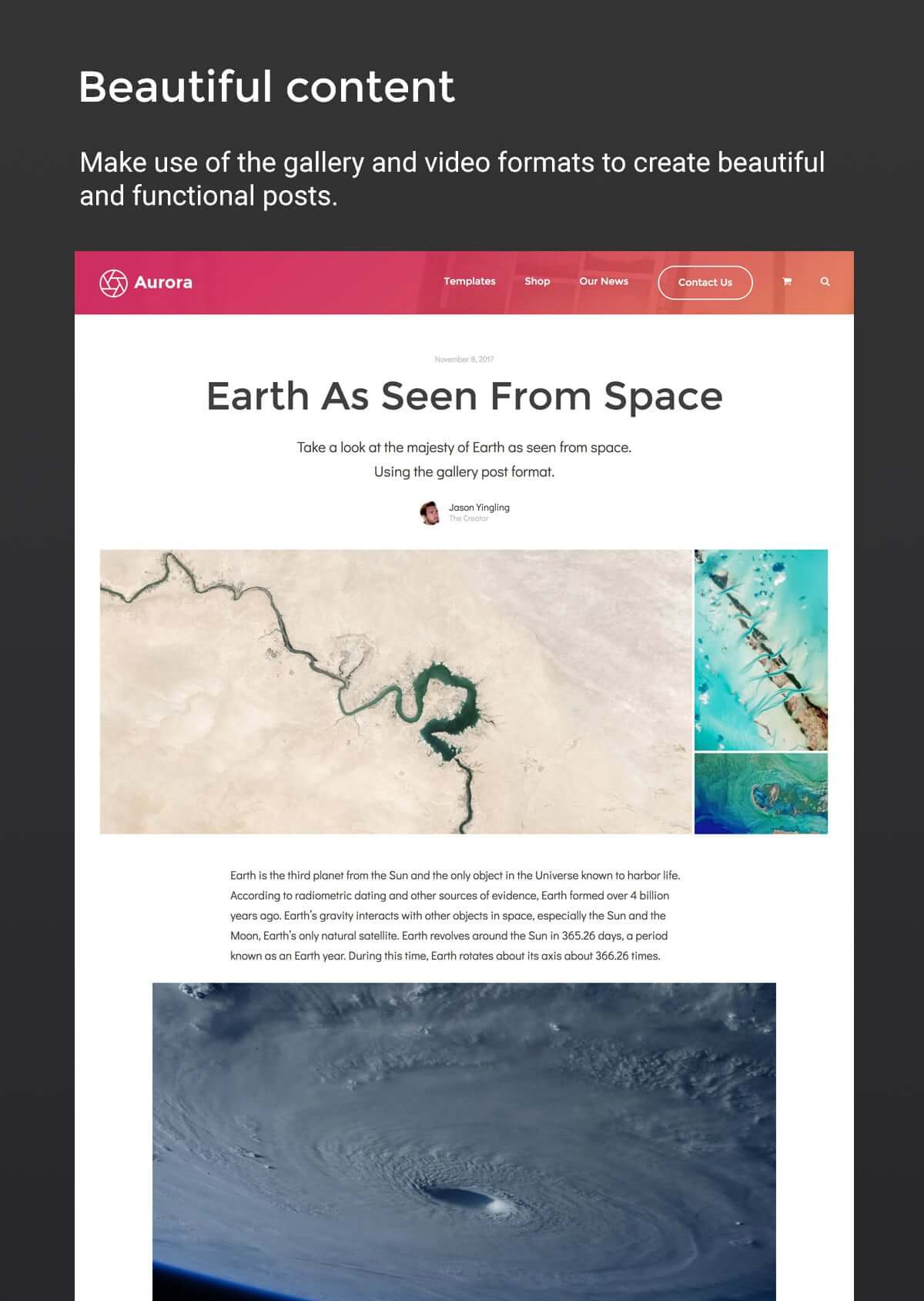A mobile phone screen showcases a sleek and minimalist design, featuring a predominantly black background with content written in elegant white text. The screen edges are framed by the device's black bezel. At the top of the screen, there is no additional information, maintaining a clean and uncluttered look.

Centered on the screen, an eyecatching red banner prominently displays a logo with the word "Aurora" next to it. Just beneath this, a navigation bar includes options such as "Templates," "Shop," "Our News," and "Contact Us," accompanied by a star icon possibly indicating a favorites feature. A search bar is also available at the top right corner, allowing users to quickly find specific content.

Below the navigation bar is a feature article on a white background, titled "Take a Look at the Majesty of Earth as Seen from Space," emphasizing the use of gallery post formats to highlight stunning visuals. The article is complemented by three captivating images from space: one showing a vibrant river, another depicting icy waters with various colorations, and a third illustrating a powerful hurricane swirling magnificently.

Accompanying these images is a descriptive paragraph that provides an in-depth narrative about the presented visuals. This setup demonstrates the platform's capability to create beautiful and functional posts using both gallery and video formats, making it an excellent tool for showcasing content.